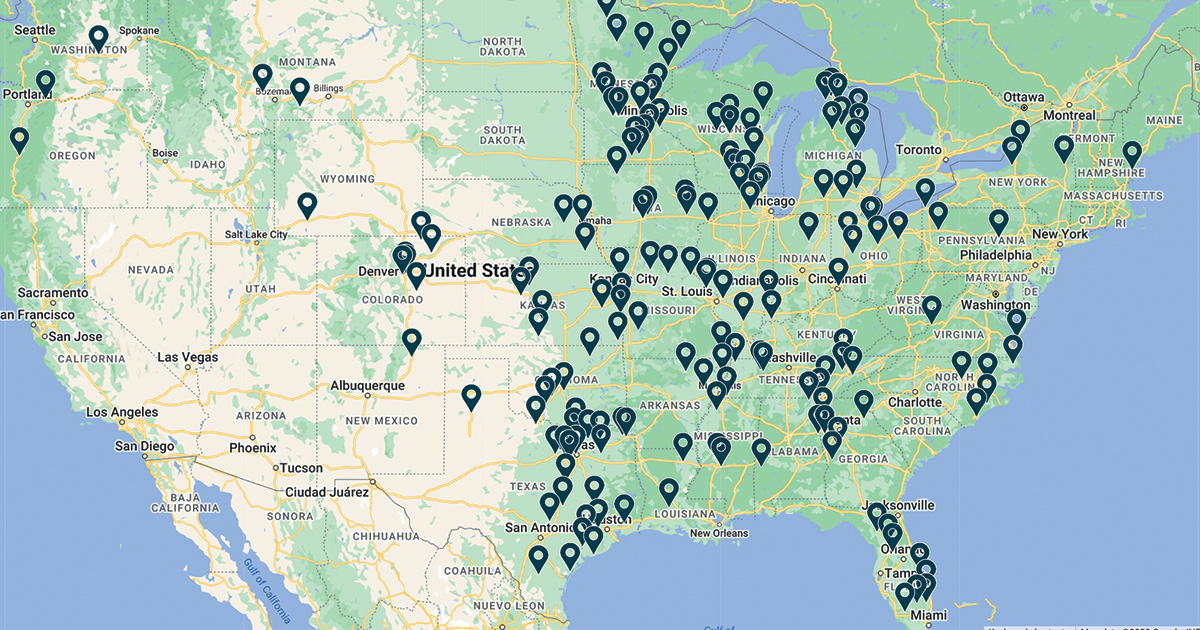This image displays a map of the continental United States, resembling a zoomed-out view from a Google Map. The map is predominantly green and devoid of a key or legend, leaving the purpose of the location markers, represented by circle-point pins, unidentified. These markers are densely situated from the Midwest to the East Coast, prominently in states like Wisconsin, Missouri, and Texas, while being entirely absent in western states such as Utah, Nevada, Arizona, and California. Similarly, northeastern states like Massachusetts, Connecticut, Rhode Island, New Jersey, Delaware, and Maryland also lack any markers. The clustering of pins east of the Mississippi River, particularly from eastern Texas to Ohio and Florida, suggests significant activity or points of interest in these areas, although the exact reason behind their placement remains unclear.